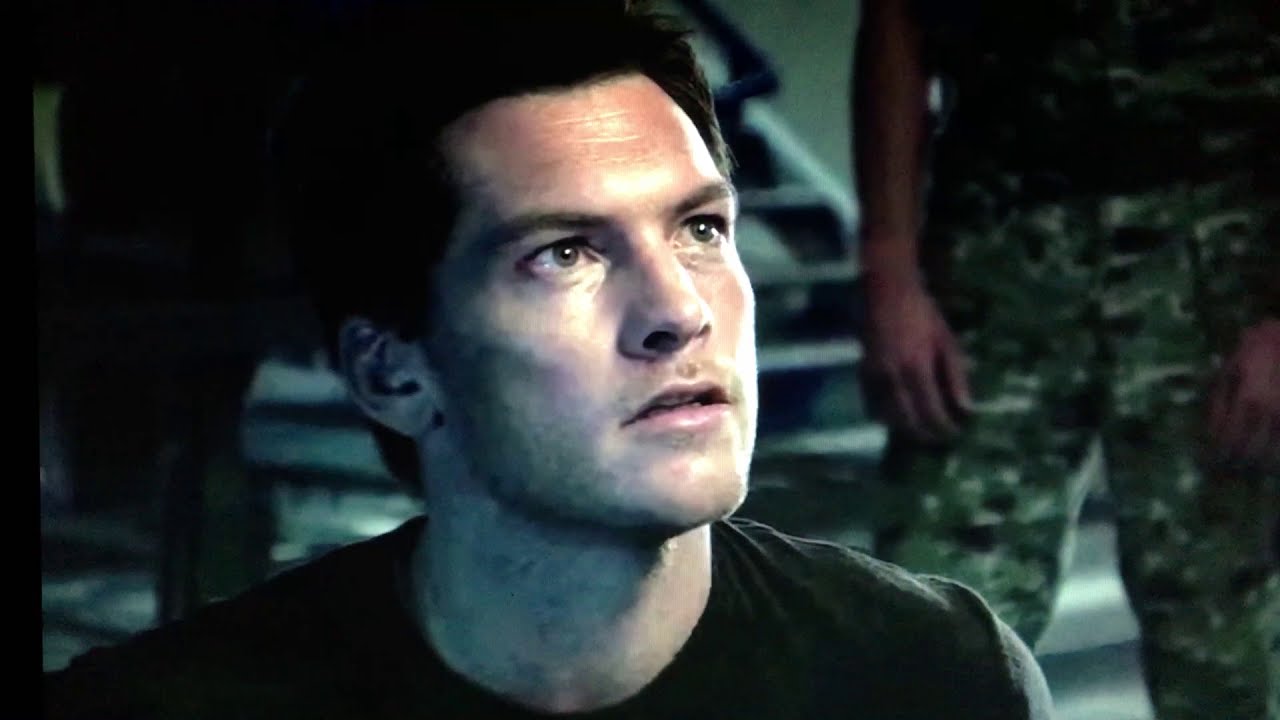The image depicts a man with short dark hair and a five o'clock shadow, dressed in a simple black t-shirt, looking up to the upper right with a concerned expression on his face. His greenish-brown eyes stand out, and his forehead appears slightly red. His mouth is partially open, revealing both his top and bottom teeth slightly. Behind him, there is another person, partially visible, dressed in army fatigues with camouflage pants, whose arms are hanging straight down. In the background, there is a blurry, barely visible staircase leading upwards, along with indistinct black shadows on the left-hand side. The man in the forefront is the main focus of the image, with light shining on his face enhancing the serious and contemplative tone of the scene.